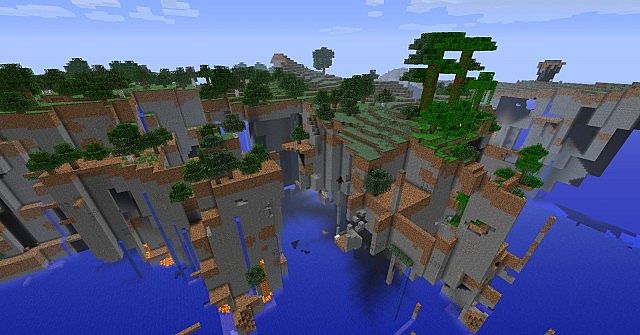The computer-generated image strongly resembles the visual style of the Minecraft game. In the background, a serene blue sky is spotted with fluffy, geometric-shaped clouds. Stretching across the middle ground are various stone buildings, all of similar size, while clusters of bushes pepper the scene, maintaining uniformity except for a notably larger tree on the right-hand side. Beyond the buildings, a lush landscape features verdant trees and towering mountains, with a tranquil body of blue water nestled below. The overall setting appears to be a fusion of forest and ocean environments, rendered predominantly in tones of green, brown, blue, and beige. Notably, the image is devoid of any human presence, further emphasizing the untouched beauty of this pixelated world.